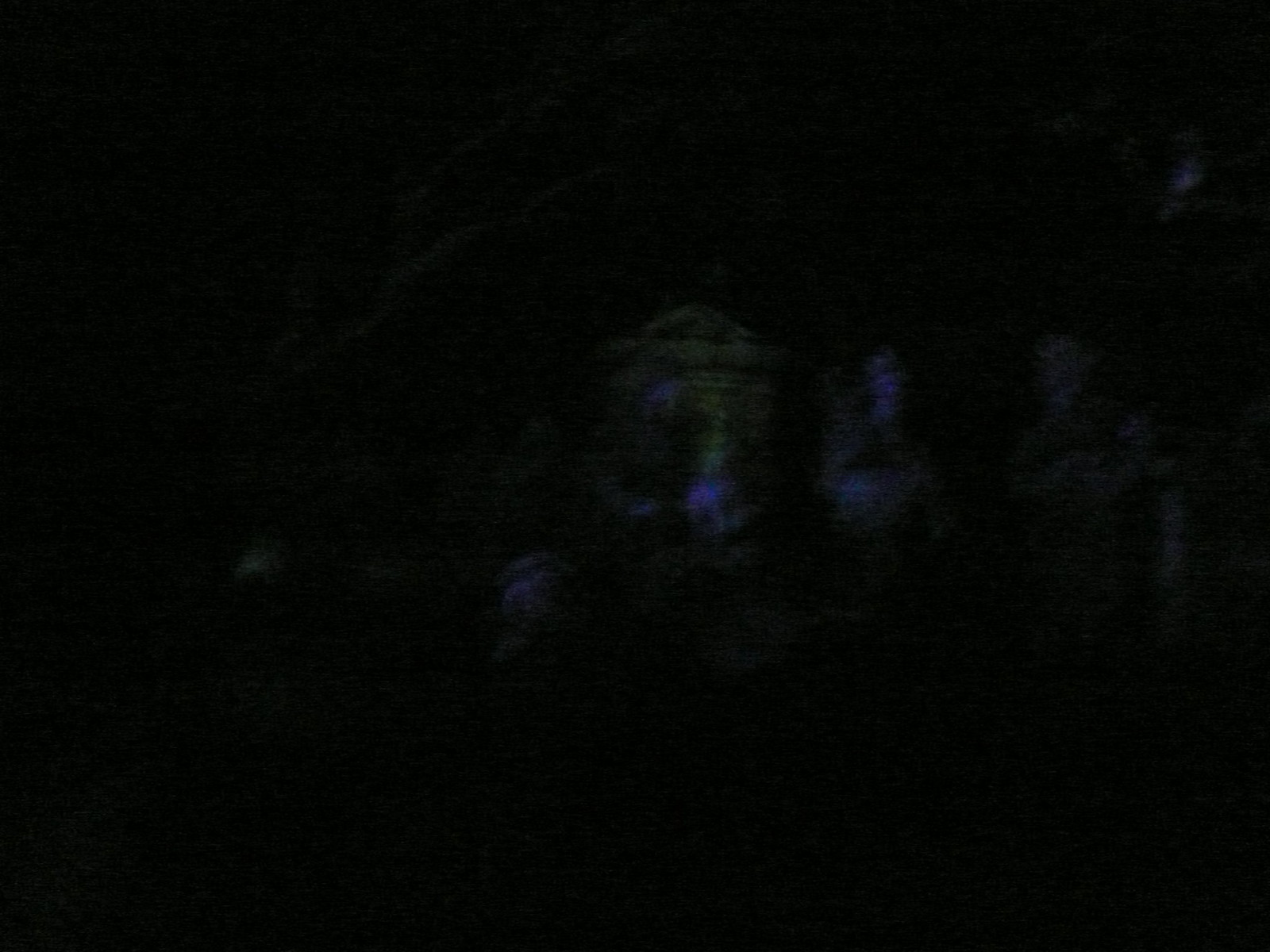The image is predominantly black, possibly taken at night or in a dark setting, rendering most details indistinguishable. However, in the center and slightly towards the right, there are faint outlines that suggest a creepy atmosphere. These include what appear to be five or six faces, characterized by white features that seem to stare directly at the camera. Surrounding these faces, there are some indistinct bodies, with visible chest and arms. Additionally, a yellowish stone structure and some branches can be seen behind these figures.

Colors and patterns are sporadically visible amidst the darkness. There is some brown and blue coloration that hints at undefined shapes, possibly forming a round circle with black dots, and a green tinge that seems to emerge from the top. Despite these slight colorations, the overall image remains overwhelmingly indistinct and eerie, contributing to its unsettling effect.